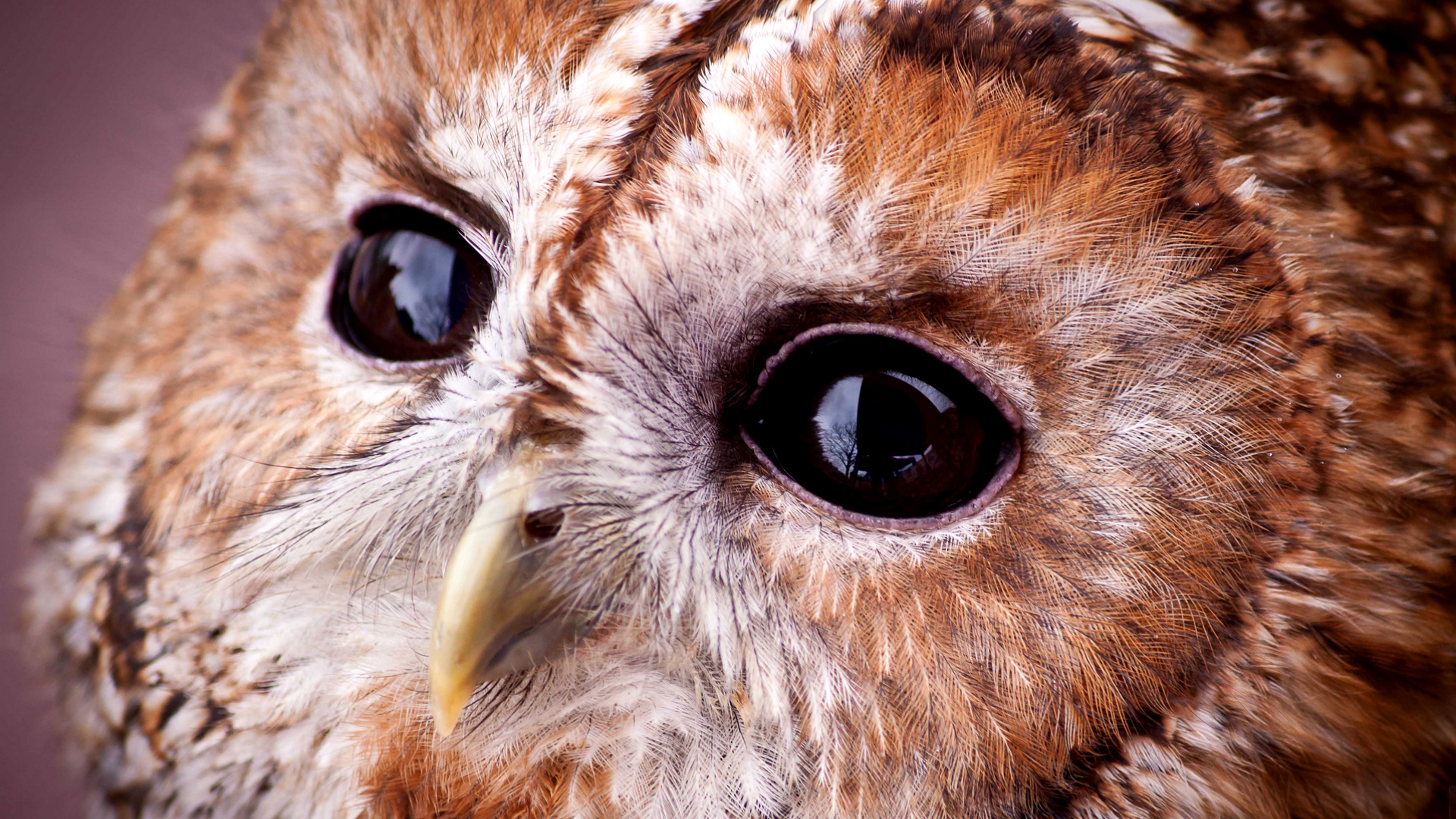This color photograph, which is not framed, signed, or dated, features a close-up of an owl set against a slightly purple background. Dominating the frame, the owl presents a mix of dark brown, light brown, and white feathers. Its face is intricately detailed: around the insides of its eyes is a ring of white, and a distinctive brown stripe runs from the top of its head down to its beak. The owl's beak is yellow at the tip, transitioning to black and gray toward its base. The owl's eyes, black and shiny with reflections of a tree and a blue sky with white clouds, add depth to its gaze. Surrounding the beak are white feathers, and the chin displays white, brown, and tan hues. Light brown feathers streak above the owl's eyes, further contributing to the rich tapestry of colors and textures on its face and body.